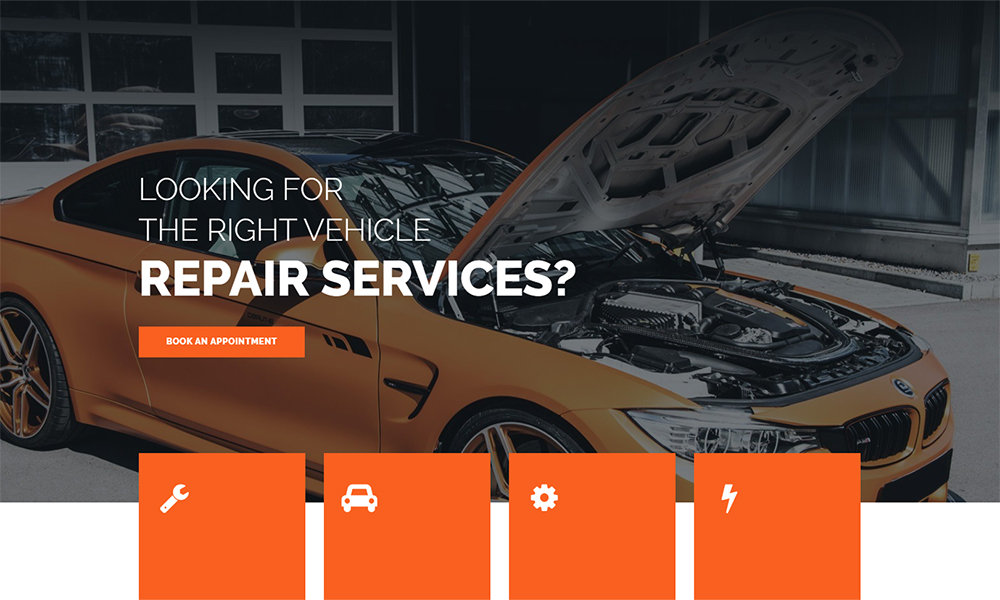**Detailed Caption:**

The image features an eye-catching orange BMW M3 with tinted windows, white interior seats, and black accents. The car is parked with its front hood open, revealing a meticulously maintained black engine with prominent black bracing. Notable exterior details include black roofing, a black front lip splitter on the bottom right, and a black grille. The BMW M3 also boasts stylish wheels, with black tires, white rims, and gold accent details.

In the center of the image, there is a prominent white text that reads, "Looking for the right vehicle, the repair services?" just above an orange button labeled "Book Appointment." Below this primary button, there are four square orange buttons, each featuring a white icon. The first button on the left displays a wrench icon, the second shows a car icon, the third features a gear lever icon, and the fourth has a lightning bolt icon.

Adding to the overall detailing, several stickers adorn the orange exterior of the car, enhancing its sporty appearance. The backdrop and layout effectively draw attention to both the vehicle and the call-to-action elements, creating a visually appealing and informative display.